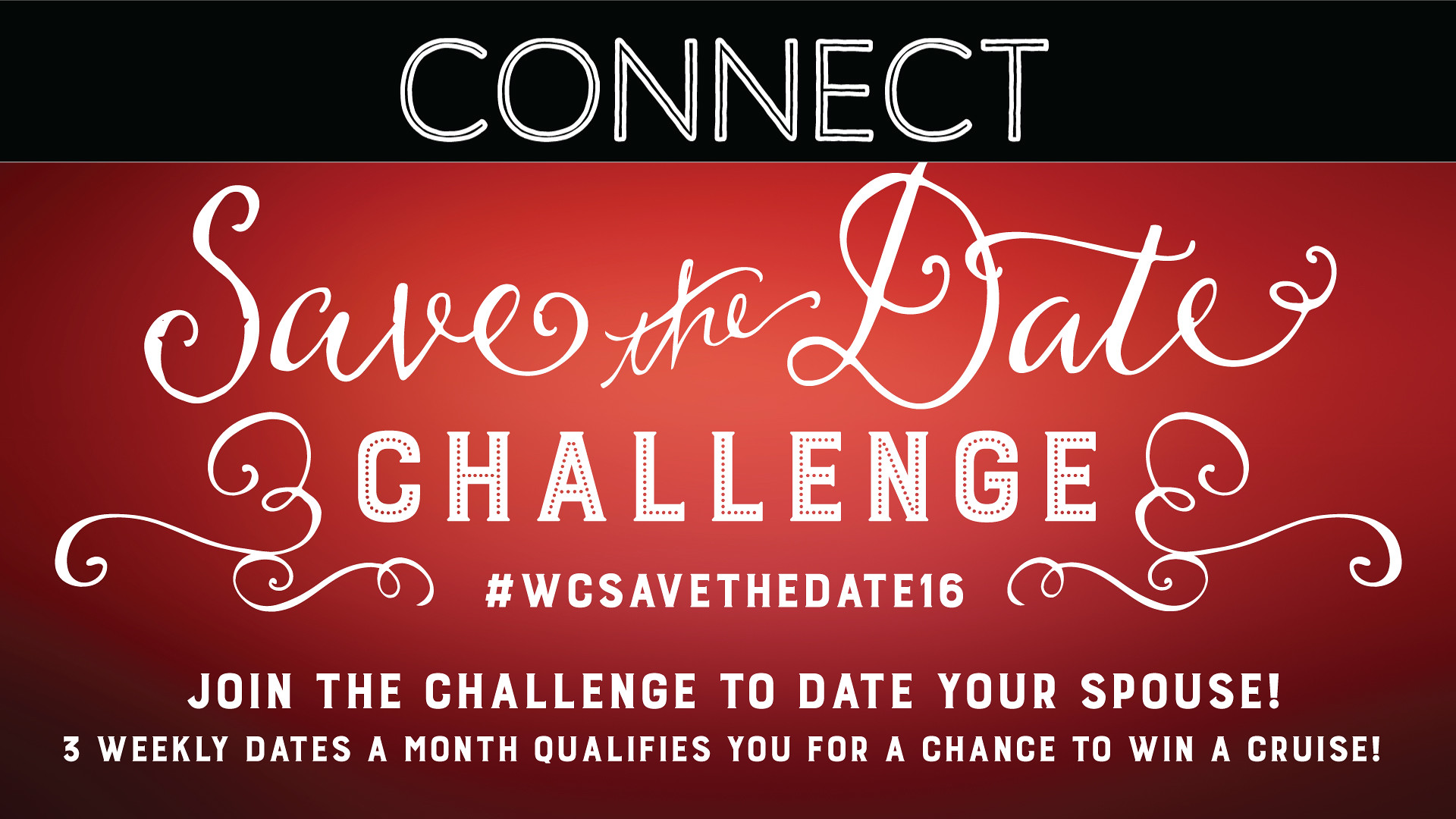This image is a promotional graphic, featuring a bold black and red background with white text. At the top, on a black bar, the word "CONNECT" is prominently displayed in all capital letters. Below it, on a red background, is cursive text that reads "SAVE THE DATE," followed by the word "CHALLENGE" in capital block letters, flanked by scroll flourishes on either side. Underneath, there is a hashtag "#WCSAVETHEDATE16." The bottom of the image reads, "JOIN THE CHALLENGE TO DATE YOUR SPOUSE. Three weekly dates a month qualify you for a chance to win a cruise." This advertisement appears to encourage couples to participate in a dating challenge for an opportunity to win a prize, potentially supporting local businesses by promoting frequent, tracked dining experiences or activities.